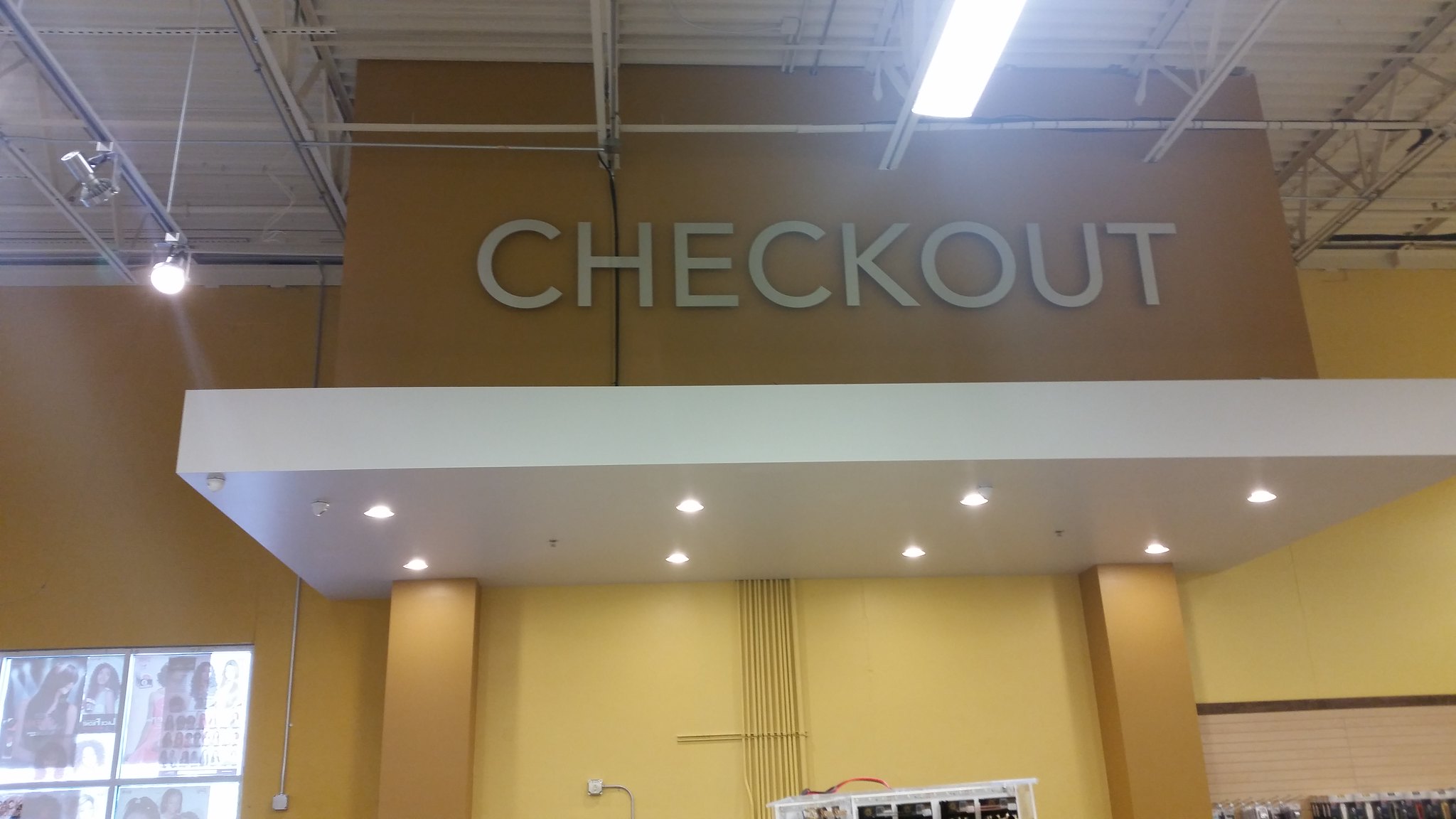The image depicts the interior view of what appears to be a large warehouse store or supermarket. The ceiling is white with visible white rafters, from which hang both long fluorescent lights and small circular spotlights, contributing to an industrial vibe. The upper part of the image showcases a mustard-colored wall prominently displaying the word "Checkout" in large white text. Below this wall, there is a white overhang featuring inset lights and noticeable indentations. Supporting the overhang are two yellow pillars, positioned on each side. On the lower left side of the wall, signs with various images of people are visible. Additionally, there is a window on the left-hand side through which green and brown colors can be seen outside, suggesting an exterior view. The overall composition focuses on the structural elements and the well-lit checkout area, framed within an otherwise nondescript space.